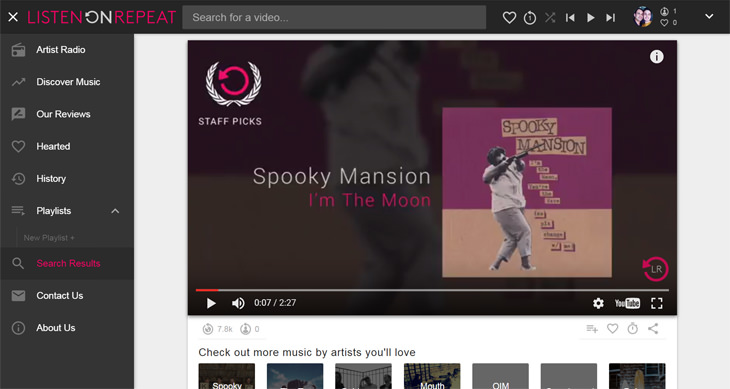This image shows a detailed homepage layout for a music streaming website. The top half-inch of the page features a solid black border spanning the entire width. Just below this, approximately two inches from the left, begins a dark gray section that extends to the middle of the page. The remaining background, extending to the right edge, is a light grayish-blue shade.

In the top left corner, a white 'X' icon is prominently displayed next to the text elements. 'LISTEN' appears in bold red, all capital letters, followed by 'on' in white, and 'REPEAT' again in red. Nearby, there is a search bar that stretches a little past the halfway mark of the page. This search bar is accompanied by a white heart icon, a refresh icon, and two arrows crossing each other like an 'X,' symbolizing repeat or shuffle functions. Additionally, there are playback controls including a reverse button, a play button, and a fast-forward button.

On the left side, there is a column featuring icons and profiles. It showcases what appears to be a profile picture of a man and a woman. Below this, a menu lists various options starting with 'Artist Radio' next to a radio icon, 'Discover Music' beside a squiggly arrow, followed by 'Hearted Songs,' 'History,' and 'Playlists.'

Following this section, a black border repeats the search icon. Next to it in pink text is 'Search Results,' and below, there are two options in white, once again on the grayish-blue background. 

In the main middle section of the page, a featured song is displayed. There is a picture relevant to the currently playing song, adorned in the top corner with a floral emblem reminiscent of Roman times. Within this emblem is a circle with an arrow pointing down, colored in pink. Under this, the section title 'Staff Picks' is shown. To the right, the song title 'Spooky Mansion' is highlighted in white text, and beneath it, another song title, 'I'm the Moon,' appears in pink text. 

Highlighted among the album covers is one featuring a distinctive design: the top half of the cover is purple, the bottom half tan. The focal point is an African-American woman holding a gun, dressed in a white shirt and tan pants.